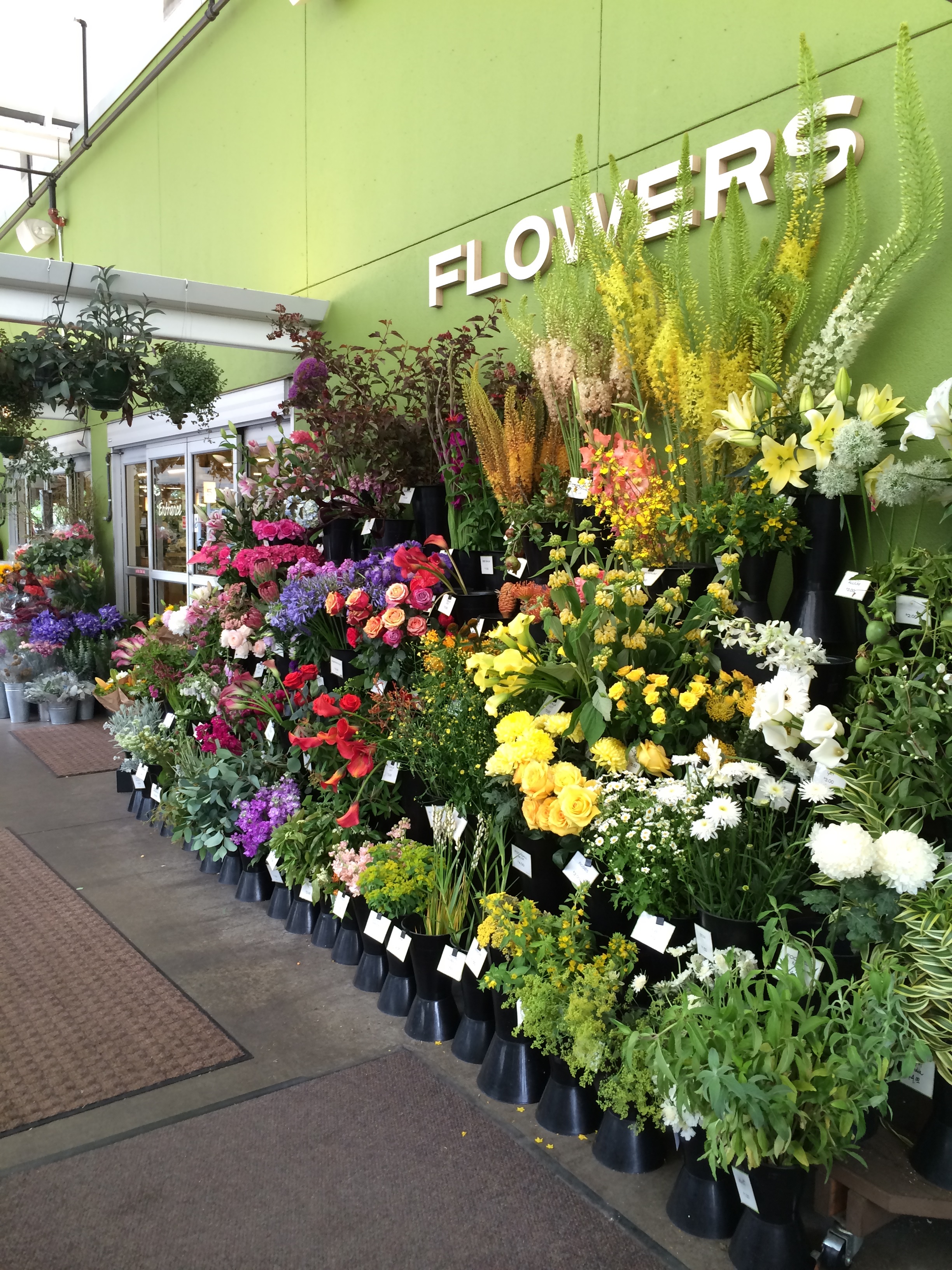The image depicts the expansive outdoor garden section of a large floral shop, distinguished by its light green façade. Prominently displayed on the wall in white letters is the word "Flowers." The shop, which resembles a wholesale establishment or possibly part of a larger market or hardware store, features rows of vibrant flowers in front of the entrance. There are five rows of flowers, varying in size, color, and type. The flowers are arranged in black pots, with taller varieties placed at the back and shorter ones in the front. Colors range from white, yellow, red, purple, and beige to light pink, among others. Next to the flower section are large glass and steel sliding doors, marking the entrance to the store. Hanging plants adorn a white support beam to the left, and mats are visible on the concrete flooring below the flower displays, indicating a well-organized and detailed presentation of the shop's floral offerings. The scene is set under a cloudy sky, adding a muted backdrop to the vibrant display.